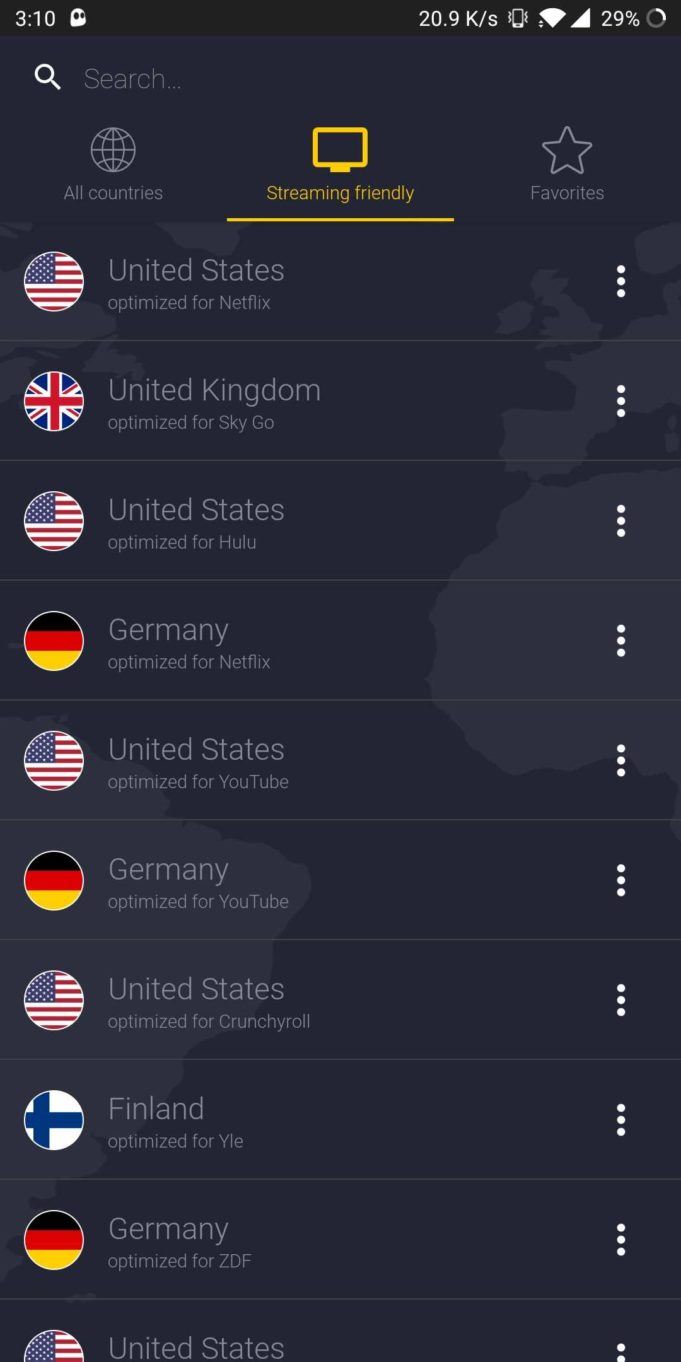Screenshot of a smartphone at 3:10 PM displaying a VPN app interface. The status bar shows full Wi-Fi and signal strength indicators, with the battery at 29%. A ghost cartoon icon is situated near the top, alongside a '20.9K per second' label, indicating data throughput. Vibration mode is turned on. 

Below the status bar, a search option is present, followed by three icon tabs: a gray globe labeled "All Countries," a yellow computer screen with "Streaming Friendly" and a yellow bar beneath it, and a gray star labeled "Favorite." 

The main section lists various countries with their respective flags within white circles on the left, and a vertical three-dot menu on the right for additional options. Each entry details which streaming service is optimized for that region. 

The dark gray background features faint outlines of world continents, including parts of Europe, Africa, North America, and South America. 

The specific entries are: 
1. United States - optimized for Netflix 
2. United Kingdom - optimized for SkyGo 
3. United States - optimized for Hulu 
4. Germany - optimized for Netflix 
5. United States - optimized for YouTube 
6. Germany - optimized for YouTube 
7. United States - optimized for Crunchyroll 
8. Finland - optimized for YLE 
9. Germany - optimized for ZDF 
10. An incomplete entry for the United States. 

This likely indicates a VPN application tailored for various streaming services across different countries.